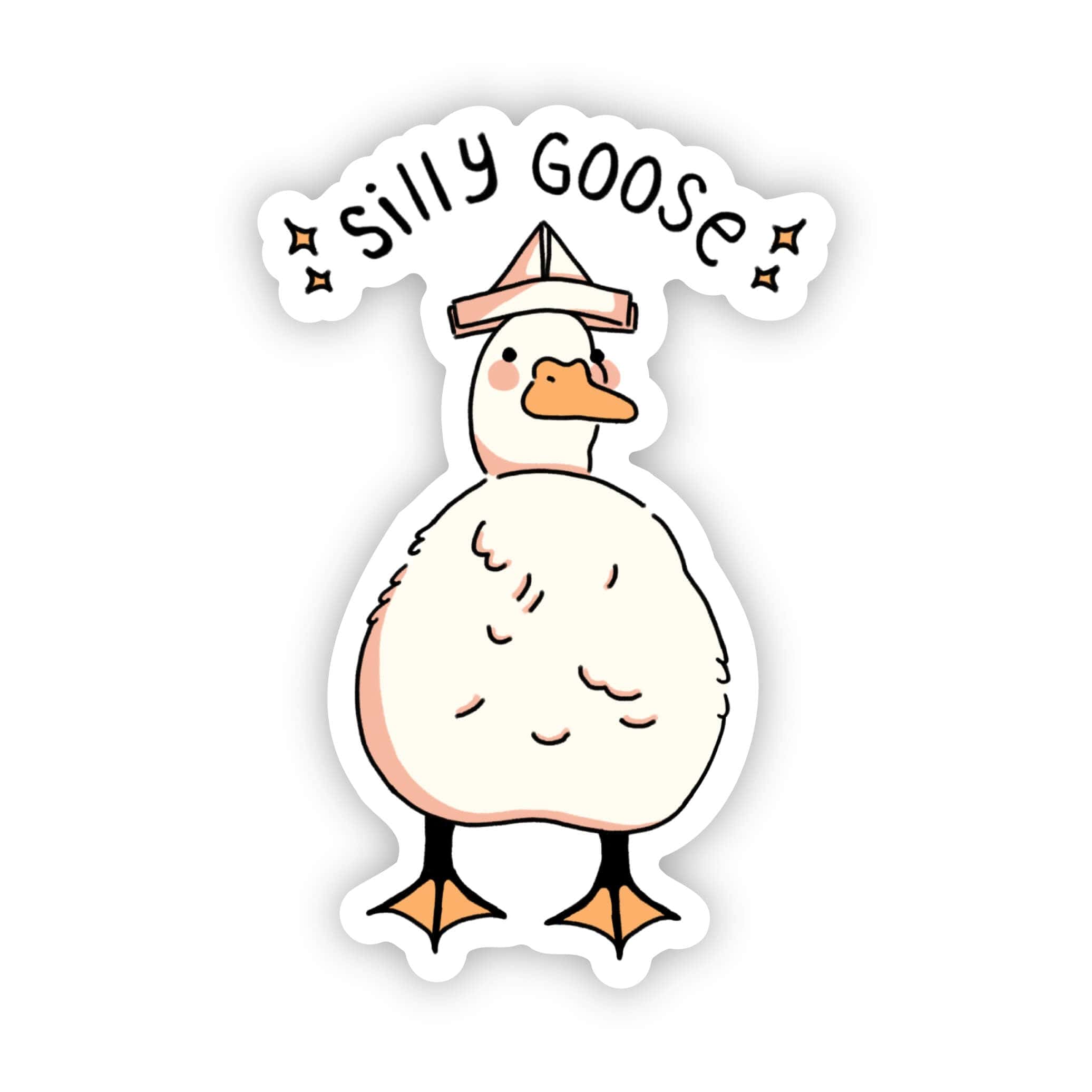This image showcases a charming sticker set against a white background. At the center of the sticker, a cartoon-style goose with black eyes, pink cheeks, and a yellow bill captivates attention. The whimsical goose, depicted with simple line drawings and limited colors—predominantly white, light pink, orangey yellow, and black—stands on its yellow webbed feet.

Perched atop the goose's head is a playful paper ship hat, reminiscent of a sailboat, adding a delightful touch of whimsy. Surrounding the goose, near the jagged-cut top edge of the sticker, are the words "Silly Goose" in black lettering. Flanking these words are two small yellow stars, one on each side, enhancing the overall playful and light-hearted tone. Designed with a childlike charm, this sticker would likely appeal to children and is perfect for adorning notebooks or other belongings, offering a delightful and inoffensive visual treat.